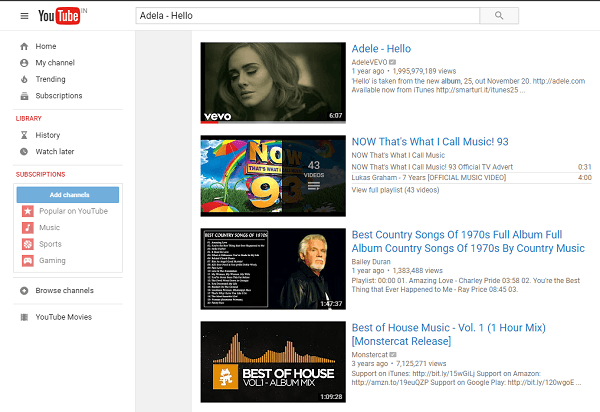Screenshot of YouTube Interface with a Search for Adele's "Hello"

The screenshot showcases the YouTube interface, which appears to have a unique look that might be specific to India or modified through a browser extension. The interface features a pane of options on the left side, including Home, My Channel, Trending, Subscriptions, History, and Watch Later. Several subscription channels are visible, such as Popular Music, Sports, and Gaming.

In the search bar, "Adella-Hello" has been entered, likely a misspelling of "Adele-Hello." Despite the typo "A-D-E-L-A-E," YouTube correctly identifies the search intent. The first video result is Adele's official "Hello" music video. The subsequent search results include a "Now That's What I Call Music" playlist, a country song playlist, and a house music mix.